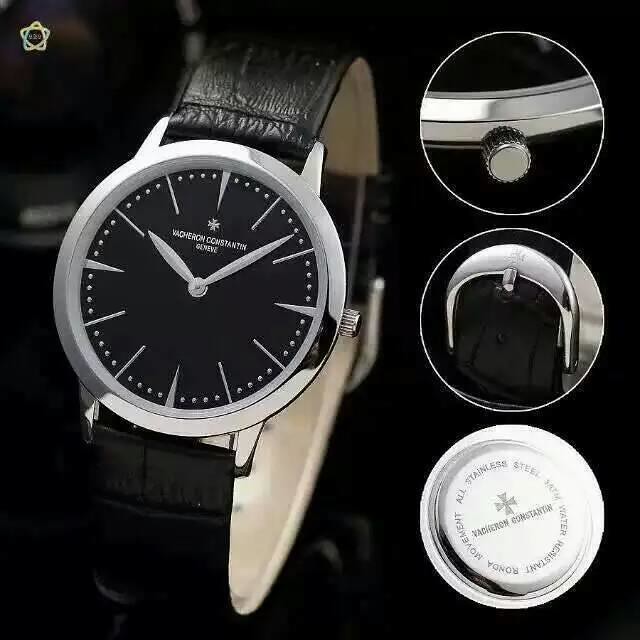This professional product photo is an advertisement showcasing a sophisticated wristwatch against a black background. The centerpiece is a watch with a black leather band, which has a cream-colored interior. The watch face is black, adorned with silver hour markers, and features silver hour and minute hands. It is not positioned upright but is slightly tilted to the right, offering a view of the bottom part of the band. The watch has a silver dial on its right side. Positioned to the right of the main image are three circular close-up shots. The top circle highlights the silver winding crown, the middle circle focuses on the silver clasp, and the bottom circle showcases the back of the watch, revealing an inscription that mentions it is made of stainless steel. The watch face has a logo resembling a cross or a plus sign and a name inscribed at the top, which is difficult to read.